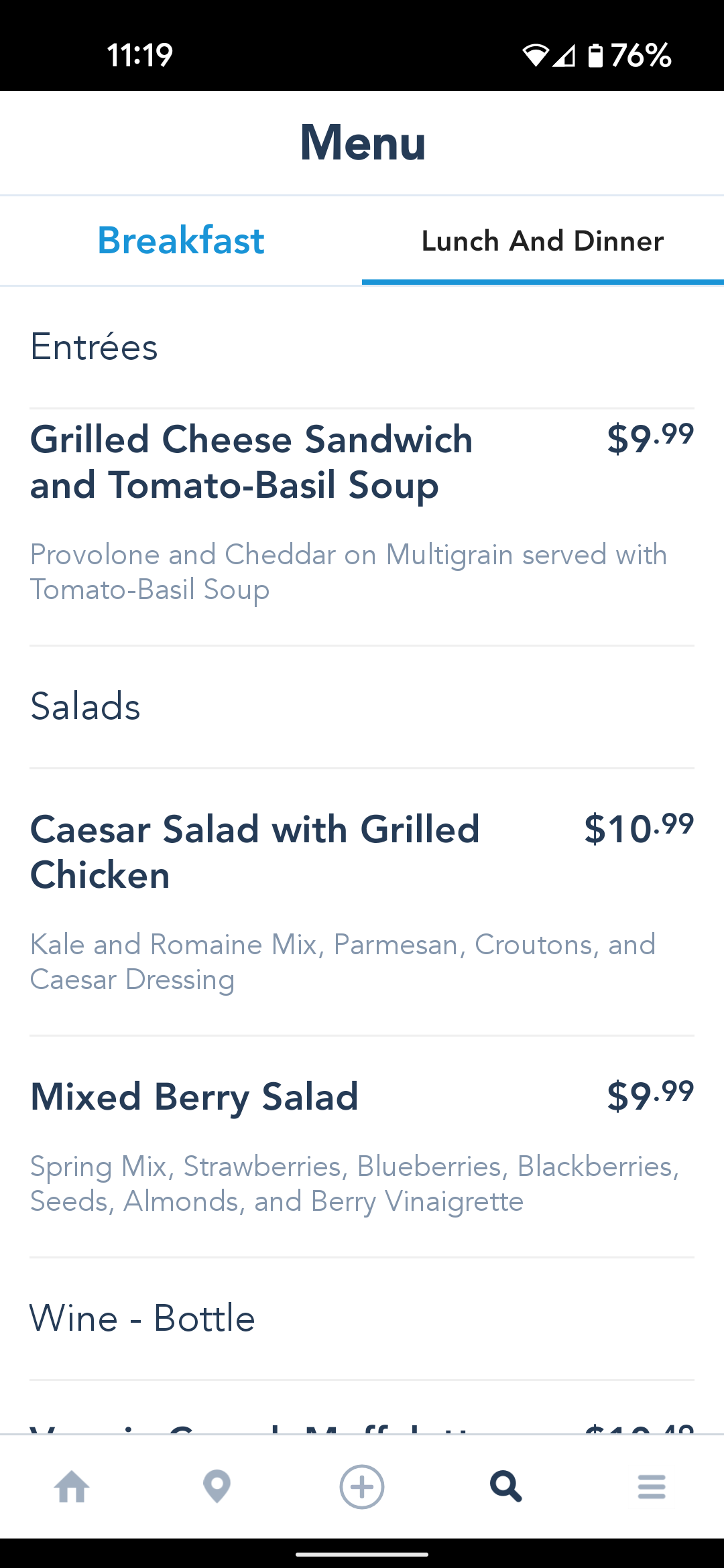This image is a screenshot of a menu taken from a cell phone using the My Disney Experience app, specifically showcasing a restaurant at Walt Disney World Resort. The screen features a white background at the top, with the word "Menu" prominently displayed in dark blue text at the center. Beneath this header, two categories are visible: "Breakfast" and "Lunch and Dinner". "Lunch and Dinner" is selected, highlighted by a black font with a blue underline, while "Breakfast" is shown in light blue font.

Directly below the category selection, the word "Entrees" appears on the left. Under the "Entrees" section, the menu lists a "Grilled Cheese Sandwich and Tomato Basil Soup" along with a brief description, and the price is displayed to the right. Following the entrees, a "Salads" section lists two items with their corresponding prices also aligned on the right.

At the bottom of the screenshot, partial text indicates a "Wine Bottle" section, though the specific selections under this category are cut off and would require scrolling to view. The footer of the app screen includes several icons for navigation: a house icon, a location icon, a plus icon, and a search icon.